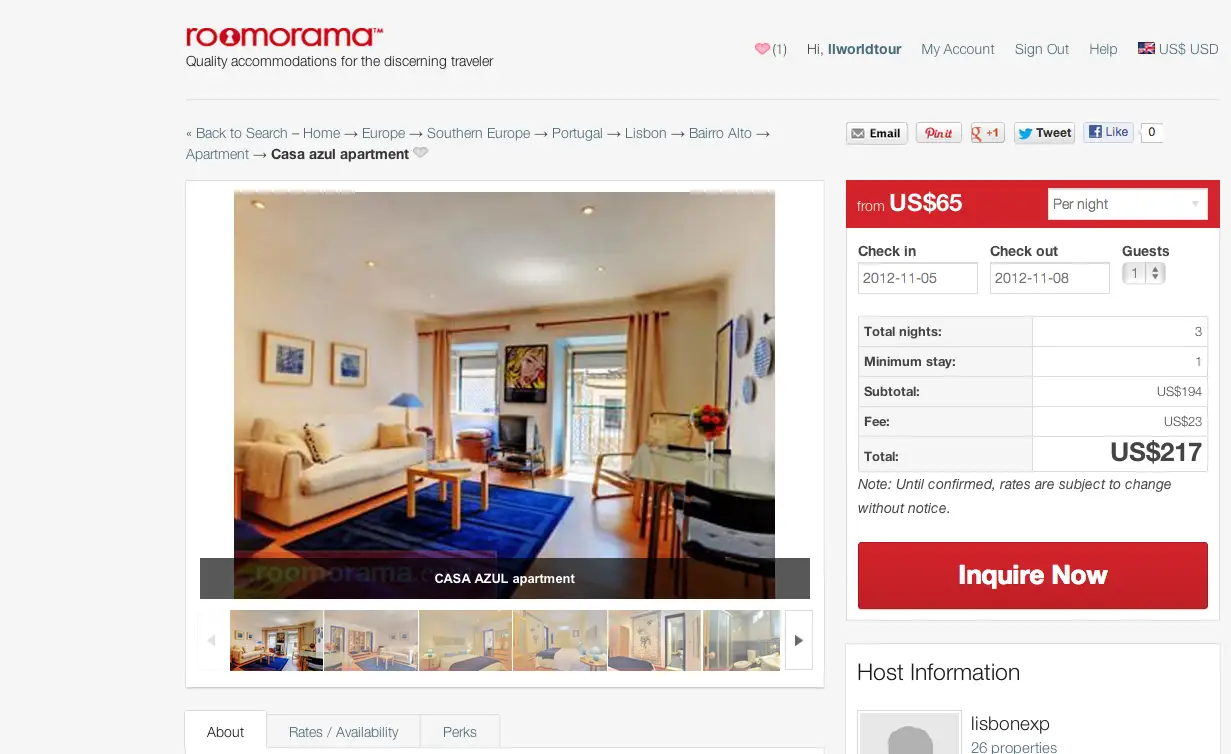**Screenshot Description: Roomorama Website Listing for Casa Azul Apartment in Bairro Alto, Lisbon**

The provided screenshot showcases a webpage from Roomorama, indicated by the all lowercase red logo featuring 'roomorama,' with the second 'O' filled in and cut out to resemble a keyhole. A small 'TM' trademark symbol is situated at the top right of the logo. Below the logo, the tagline "quality accommodations for the discerning traveler" is displayed in black text.

In the visible navigation path, the breadcrumb trail reads "back to search - home > Europe > Southern Europe > Portugal > Lisbon > Bairro Alto > Apartment > Casa Azul apartment," with "Casa Azul apartment" highlighted in bold. Adjacent to the apartment name, there is a light gray heart icon indicating it can be clicked to favorite the listing.

The primary image depicts a cozy living room area of the Casa Azul apartment. The room features beige-white walls and recessed ceiling lighting with five visible bulbs. The wall is adorned with two framed artworks in light brown frames, showcasing images with dominant dark blue tones.

The living area includes a beige couch with a blanket draped over the left armrest and a couple of beige throw pillows. To the right of the couch stands a lamp with a blue lampshade. The floor is covered by a deep royal blue rug, upon which a small four-legged coffee table sits. A window and partially visible door provide a view of the neighboring apartment.

The room is decorated with a large art piece resembling a Lichtenstein painting of a woman. Additional decorations include blue plates mounted on the right wall. A small dining table with a black chair and a small flower arrangement adds to the homey ambiance. There are also various indistinguishable objects on the floor, adding character to the space.

Overall, the Casa Azul apartment listing on Roomorama promises a well-decorated, inviting living environment for travelers looking to stay in the historic Bairro Alto district of Lisbon.